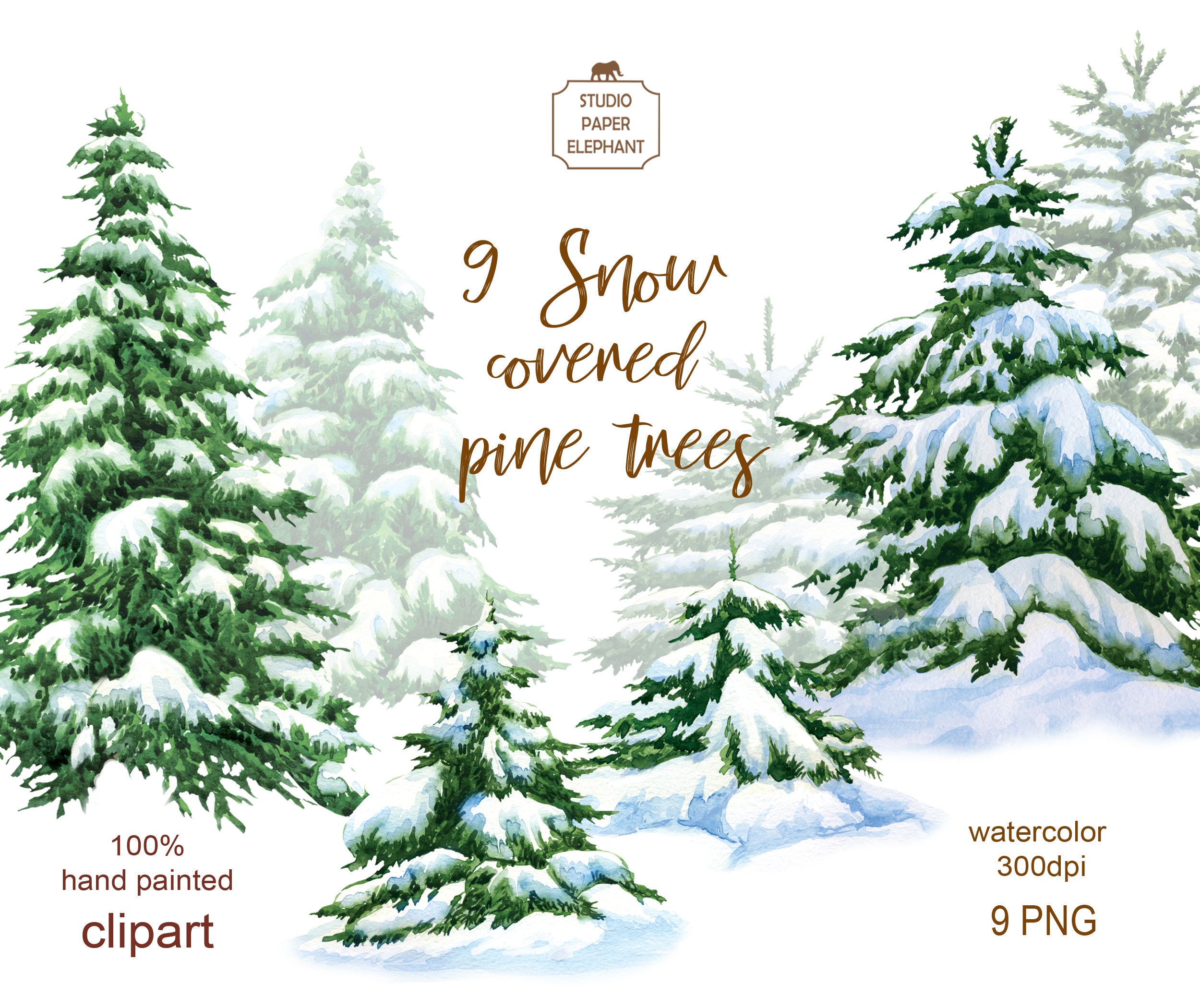This is a square image featuring a white background. At the center top, the text "Studio Paper Elephant" is outlined in brown and accompanied by a brown silhouette of an elephant walking to the right. Below this, in brown script, it reads "Nine snow-covered pine trees." The artistic content is dominated by green pine trees heavily laden with snow. In the foreground, a tall pine tree stands on each side, flanking two smaller trees in the middle. In the background, three more trees - tall, medium, and small - appear more faded. The scene depicts a wintery setting, with snow blanketing the ground and the branches. The bottom left corner states "100% hand-painted clip art" while the bottom right corner reads "Watercolor 300 DPI 9 PNG."